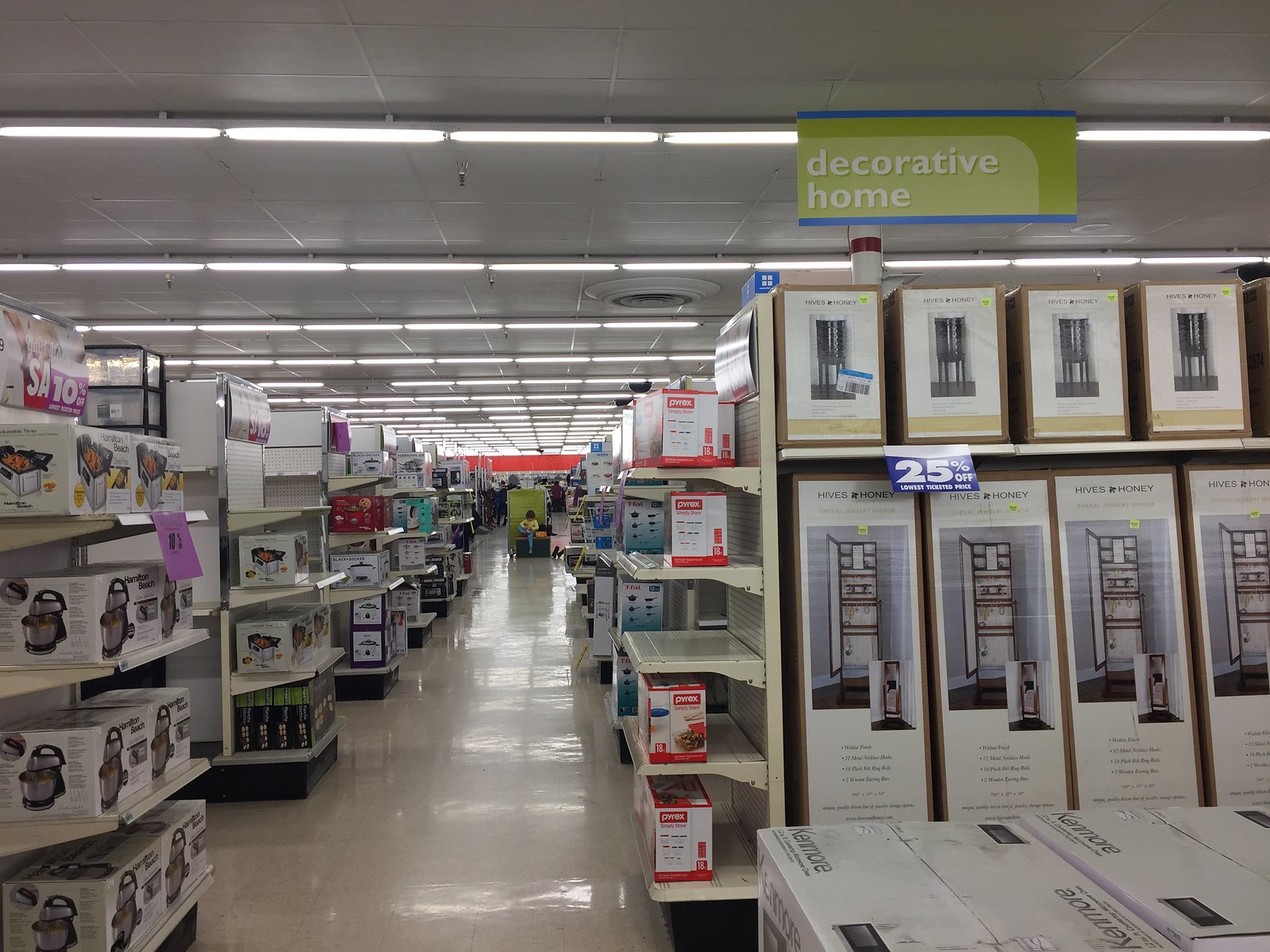The image is a color photograph taken inside a large department store, reminiscent of a Walmart or Target. The floor, made of concrete or stone tile, displays the reflections of fluorescent lighting that runs horizontally along the ceiling. In the upper right-hand corner, there's a green and blue banner that reads "Decorative Home," advertising a 25% off sale. To the right side in the foreground, there are standing refrigerators or cabinets, while numerous shelves on both sides of the aisle are stocked with various home products, including a visible crock pot on the left side. The photograph depicts a perspective moving back into a central display, with the far end of the store featuring a red strip on the wall. Fire alarm sprinklers and additional lighting fixtures are visible on the ceiling, contributing to the overall brightness of the store environment.